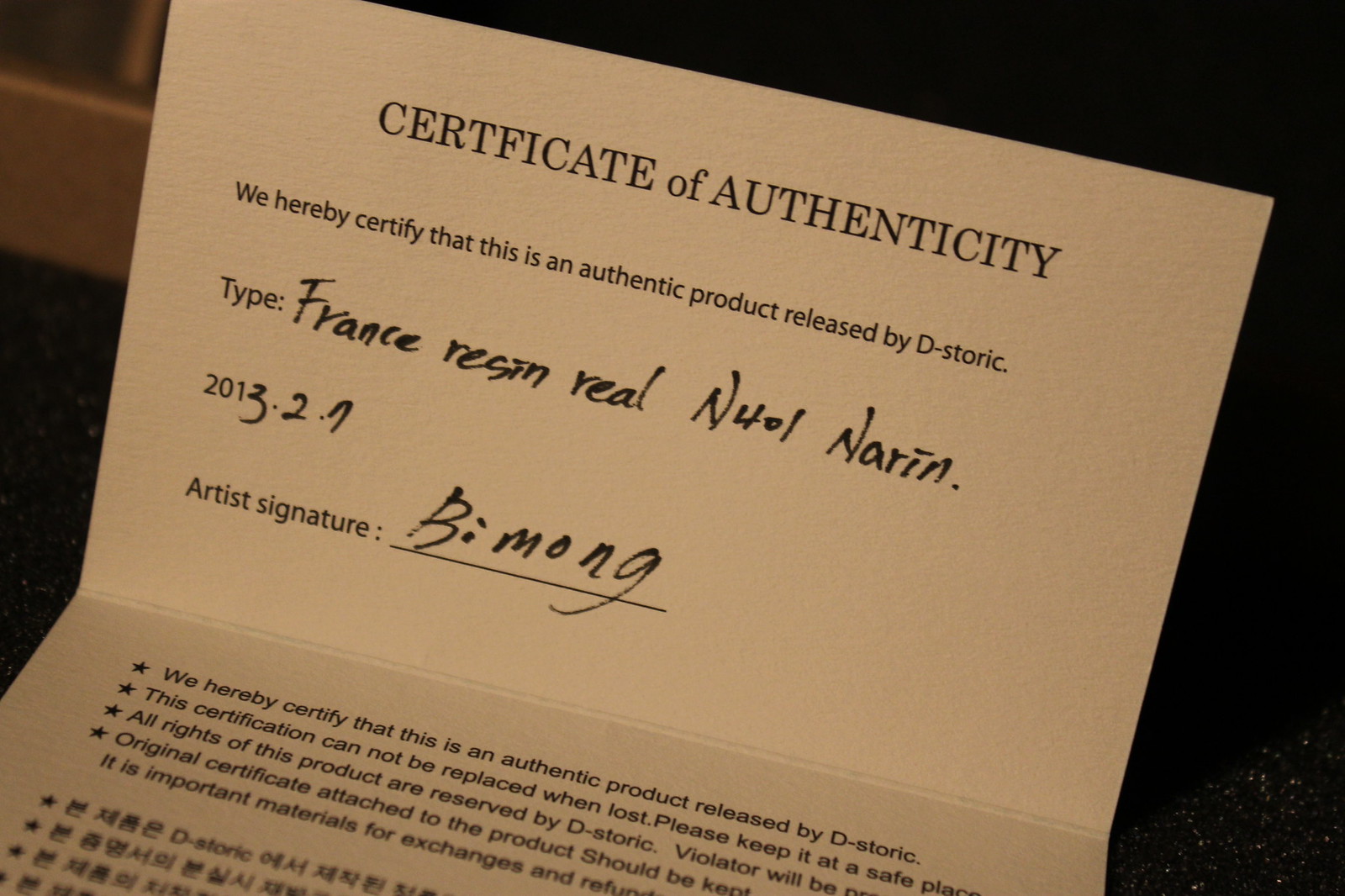The image is a photograph of a folded piece of paper labeled "Certificate of Authenticity" positioned on a slant from the upper left to the center right. The background is predominantly black with a hint of a brown table edge visible at the top left corner, suggesting the use of a flash. The certificate, printed in dark ink on a light brown paper, certifies an authentic product released by D-Storic and contains the following details: type "France, resin, real," with the code "N-401 Narin," and the date "2013-2-7." It includes an artist's signature by "BMONG" (handwritten as B-I-M-O-N-G). The lower section repeats the certification statement, noting that it cannot be replaced if lost and advising to keep it in a safe place. Additional instructions mention that the original certificate should be attached to the product and that it is important material for exchanges. This information is supplemented by a series of bullet points, some of which are translated into Chinese characters. However, parts of the text are cut off and not fully visible.